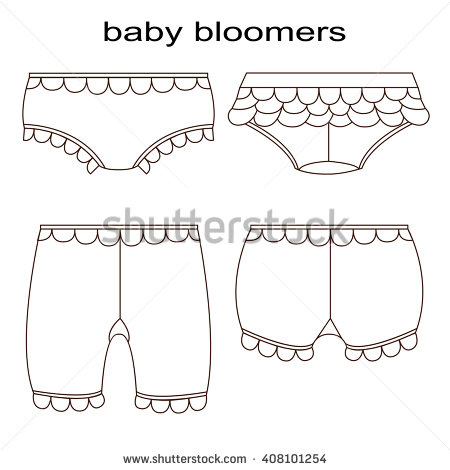This image, sourced from Shutterstock, features a clean, simple white background with the words "baby bloomers" prominently displayed at the top in lowercase black font. Below this title are four distinct line drawings representing various styles of baby bloomers. Each drawing is rendered in black ink, outlining the waist, leg holes, and decorative frills in minimalist detail. The top left illustration showcases modest brief-like bloomers with frills bordering the waist and leg openings. The top right features a slightly less modest pair with more pronounced layers of frills around the band and leg areas. On the bottom left, the bloomers extend to mid-thigh, marked by frills at the waist and leg openings, representing the most modest style. The bottom right image depicts a shorter, yet still modest pair, characterized by similar frill placement. The center of the image subtly displays "www.shutterstock.com" in a gray font, offering a clear, straightforward depiction of these ornate, but simply drawn, baby garments.